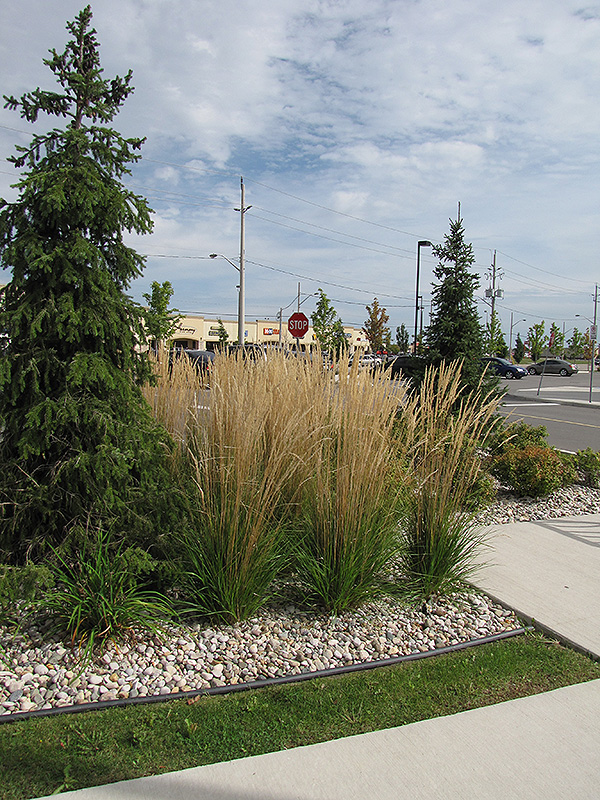This photograph, taken outdoors, captures an intricately landscaped area. At the bottom of the image is a white sidewalk, which angles upwards and widens towards the right side of the frame. Directly above this sidewalk is a neat, rectangular patch of lush green grass. Just beyond this is a strip of black mulch, which provides a striking contrast to the array of white stones that follow. Embedded within the white stones are various plantings, adding vibrant life to the scene.

On the left side of the photograph stands a fir tree, its verdant needles creating a natural focal point. Surrounding the base and extending to the right of the tree are several tall ornamental grasses. The grass directly in front of the fir tree is shorter and uniformly green, while the others are taller with a gradient of green at the bottom and a wheat color at the top, indicating seasonal change.

In the background, a stop sign is partially obscured by the ornamental grasses. Beyond the sign, the upper portion of a beige building can be seen against the sky. The sky is a soft blue, scattered with numerous white clouds that add depth and texture to the scene. The combination of natural elements and human-made structures creates a harmonious and detailed landscape.